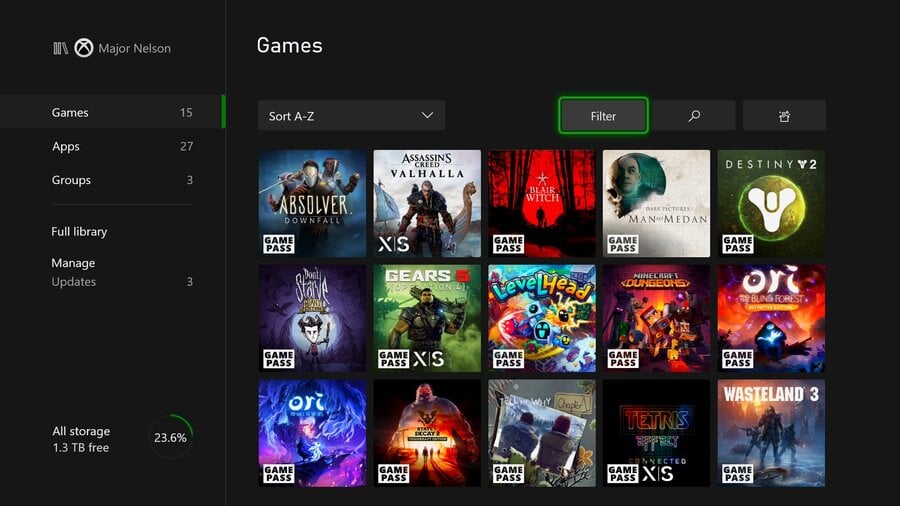The web page features a sleek, black background and is organized into three horizontal rows showcasing various video games. In the upper left-hand corner, a white circle encloses the logo and name "Major Nelson." Below this is a vertical menu in white text, listing several options: Games, Apps, Groups, Full Library, Manage Updates, and at the very bottom, All Storage. The Games option is highlighted, showing the number 15 next to it. Apps indicates 27, Groups show 3, and Manage Updates reveals 3 updates available. At the bottom, the All Storage section denotes 1.3 TB free, with 23.6% of storage used.

The rows of games are displayed with square thumbnail images, each bearing the title and cover art of the game. The first row includes games such as Absolver: Downfall, Assassin's Creed: Valhalla, Blair Witch, Man of Medan, and Destiny 2, among others.